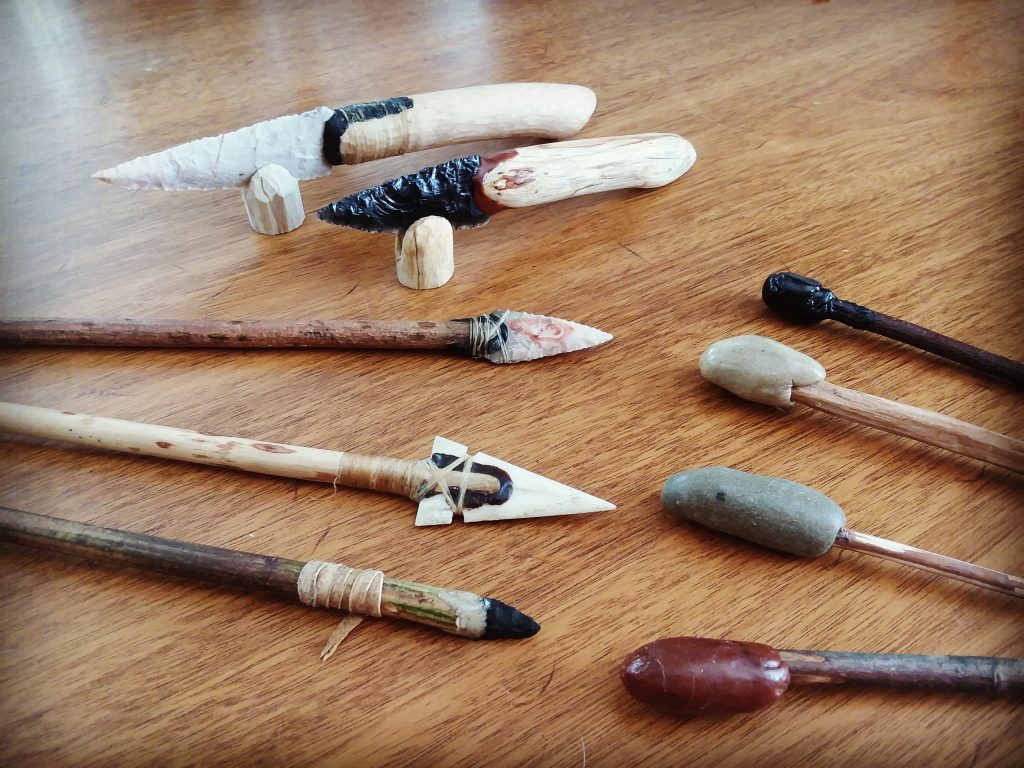This close-up indoor photograph showcases a detailed collection of Native American artifacts arranged on a wooden table. On the right side, four distinctive blunt instruments, possibly traditional drum beaters, are neatly lined up. These drum beaters, each unique in design, seem to lack the typical fur or skin wrapping but may serve varied cultural purposes. To the left of these beaters, there are three arrows, each different in appearance yet crafted with precision. Just above these arrows, in the upper left corner of the table, two primitive knives rest on small stands. These knives feature intricately chipped stone blades and bone handles, exhibiting a sophisticated blend of form and function. The overall color palette of the items is primarily tan, with one handle in black and one stone tip displaying a striking rose red. The careful arrangement and craftsmanship of these tools provide a window into the rich heritage and skilled artistry of Native American cultures.